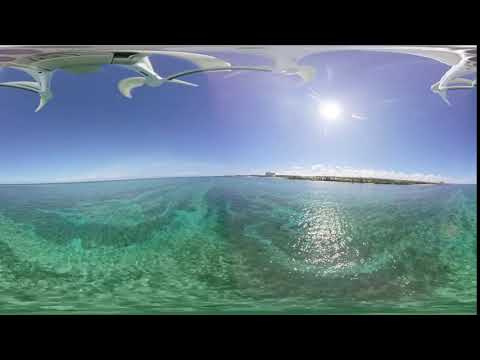This image is a panoramic photograph captured using a drone, providing an aerial view of an expansive body of water. The water displays a mesmerizing mix of teal, green, and blue hues with visible swirls, creating a sea glass appearance. The surface is wavy, suggesting tidal movement. Above, the sky is a clear, light blue, with a few wispy clouds near the horizon. The bright midday sun is prominently visible in the top-right corner, casting a radiant reflection on the water below. 

The white drone, seen distorted due to the fisheye lens effect, hovers in the upper portion of the photograph. Its propellers and pointed edges are stretched across the image, adding a dynamic element. At the horizon, a distant landmass with lush green vegetation and white sandy beaches is visible. Scattered through the water are occasional gray rocks, and the clarity of the water allows glimpses of the sandy bottom and underwater vegetation. No text is present in the image, maintaining a pure visual focus on the natural scene.